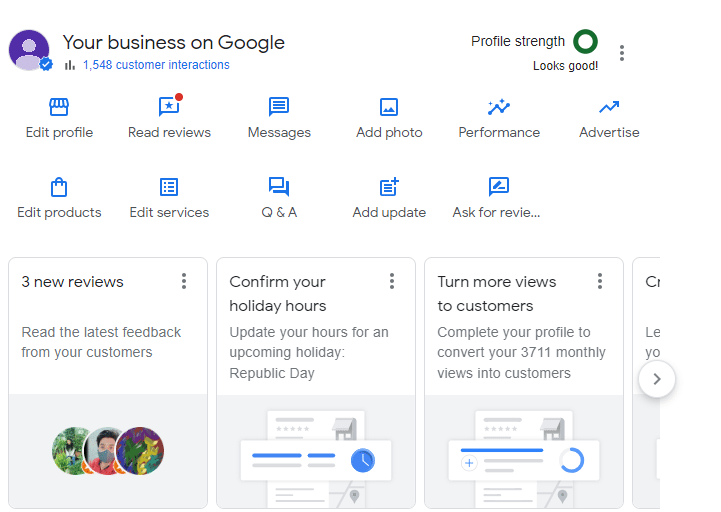The image captures a section of a website interface primarily set against a white background. At the top center, there's a prominent round purple circle, followed by a lighter purple circle representing a head, and below, a third circle signifying the shoulder area. Adjacent to these circles, there's a blue circle with a white checkmark inside.

To the right of these graphics, bold black text reads, "Your Business on Google," with "G" capitalized. Directly below, a blue text displays "1,548 customer interactions."

Further down, the phrase "Profile Strength" appears next to a green circle with a white center, accompanied by the text "Looks good." Near this element, there are three vertical dots symbolizing additional options.

Below this section, blue graphic icons accompany black text options including "Edit Profile," "Read Reviews," "Messages," "Add Photo," "Performance," "Advertise," "Share Products," "Edit Services," "Q&A," "Add Update," and "Ask for a Review."

The lower section of the page is divided into three panels. The first panel shows "Three New Reviews," prompting the user to read the latest feedback from customers. The second panel encourages the user to "Confirm Your Holiday Hours" and suggests updating hours for an upcoming holiday, notably Republic Day. The third panel highlights a call-to-action: "Turn More Views to Customers," advising the user to complete their profile to convert "3,711 monthly views into customers." A right-facing arrow inside a circle is present, possibly indicating a link or further action.